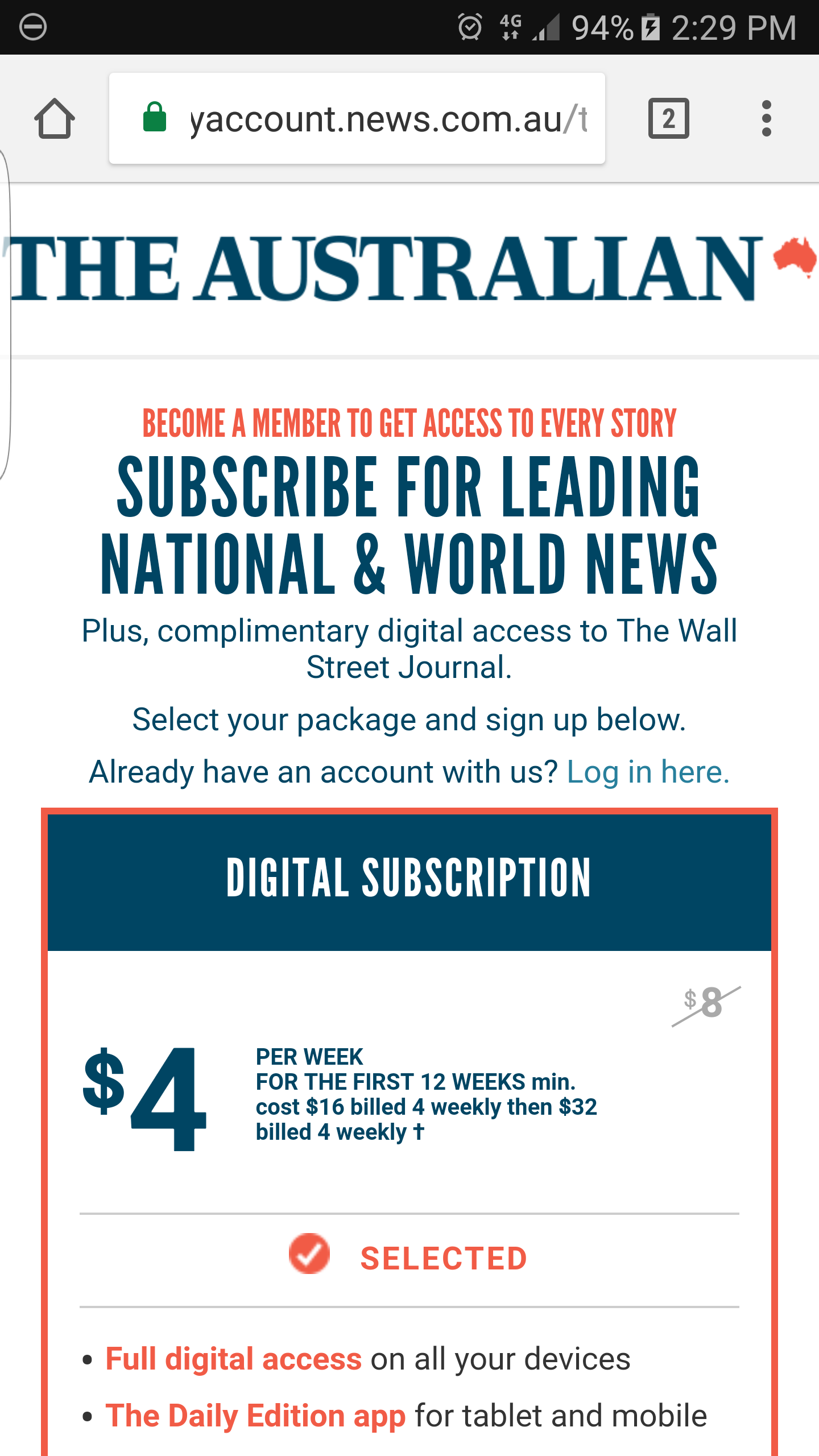The image displays a screenshot of a news website, specifically "The Australian." In the upper right-hand corner, the device's battery is shown at 94% with an almost full battery icon indicating it is charging, and the time is displayed as 2:29 PM. 

Centered prominently on the page in large print is the title "The Australian." Below, a message invites users to become members to gain access to every story, with a subscription offering leading national and world news. It also mentions complimentary digital access to The Wall Street Journal and provides a prompt to select a subscription package, sign up, or log in if the user already has an account (the log-in link is highlighted in a distinct blue shade).

Further down, a red-bordered box is visible with the text "Digital Subscription." Initially, the price is listed as $8, but this amount is crossed out. Instead, a promotional offer of $4 per week for the first 12 weeks is highlighted, specifying a minimum cost of $16 billed weekly for the first 12 weeks, and then $32 billed weekly thereafter. A red circle with a white checkmark inside it and the word "Selected" confirms the choice. Below this, two bullet points outline the benefits: full digital access on all devices, and access to the daily edition app for tablets and mobiles.